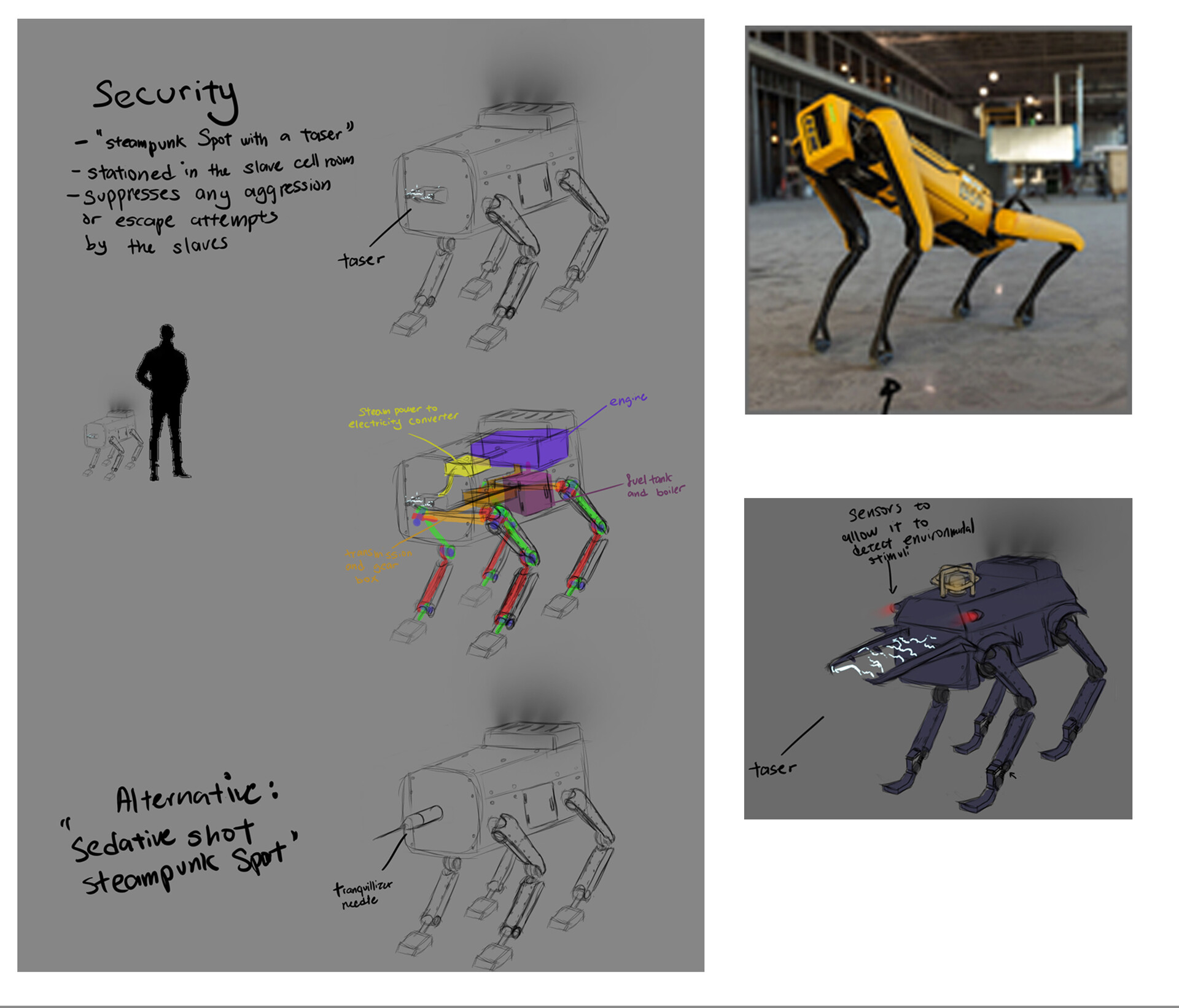The image consists of a detailed schematic and artistic renderings of a steampunk-inspired four-legged robot. The image is divided into three sections:

1. **Left Section**: Dominated by a gray background, at the top-left, there's handwritten black text reading "security." Below, it states "steampunk spot with a taser stationed in the slave cell room" and notes that the robot "suppresses any aggression or escape attempts by the slaves." This section features three drawings of the robot, resembling a rectangular box on four legs. Annotations indicate various internal components: the engine labeled in blue, the fuel tank and boiler in purple, and the steam power to electricity converter in yellow.

2. **Middle Section**: Presents a colored version of the robot's schematic. This detailed illustration highlights specific parts with distinct colors such as red, green, purple (for the engine), and yellow (for the electricity converter). It includes a standing man for scale, showing that the robot reaches up to his hip, indicating it's fairly small.

3. **Right Section**: Contains two smaller images framed against a gray background. The upper one is a rendering of what the actual robot might look like, depicted in yellow and black, with some text that's hard to decipher due to its scribbled nature. The lower box features another sketch of the robot, along with more textual information referring to an "alternative sedative shot."

Overall, the combined sections provide an in-depth look at this steampunk-themed, security-oriented robot’s design and functionality, hinting at its purpose in maintaining order within a confined space.